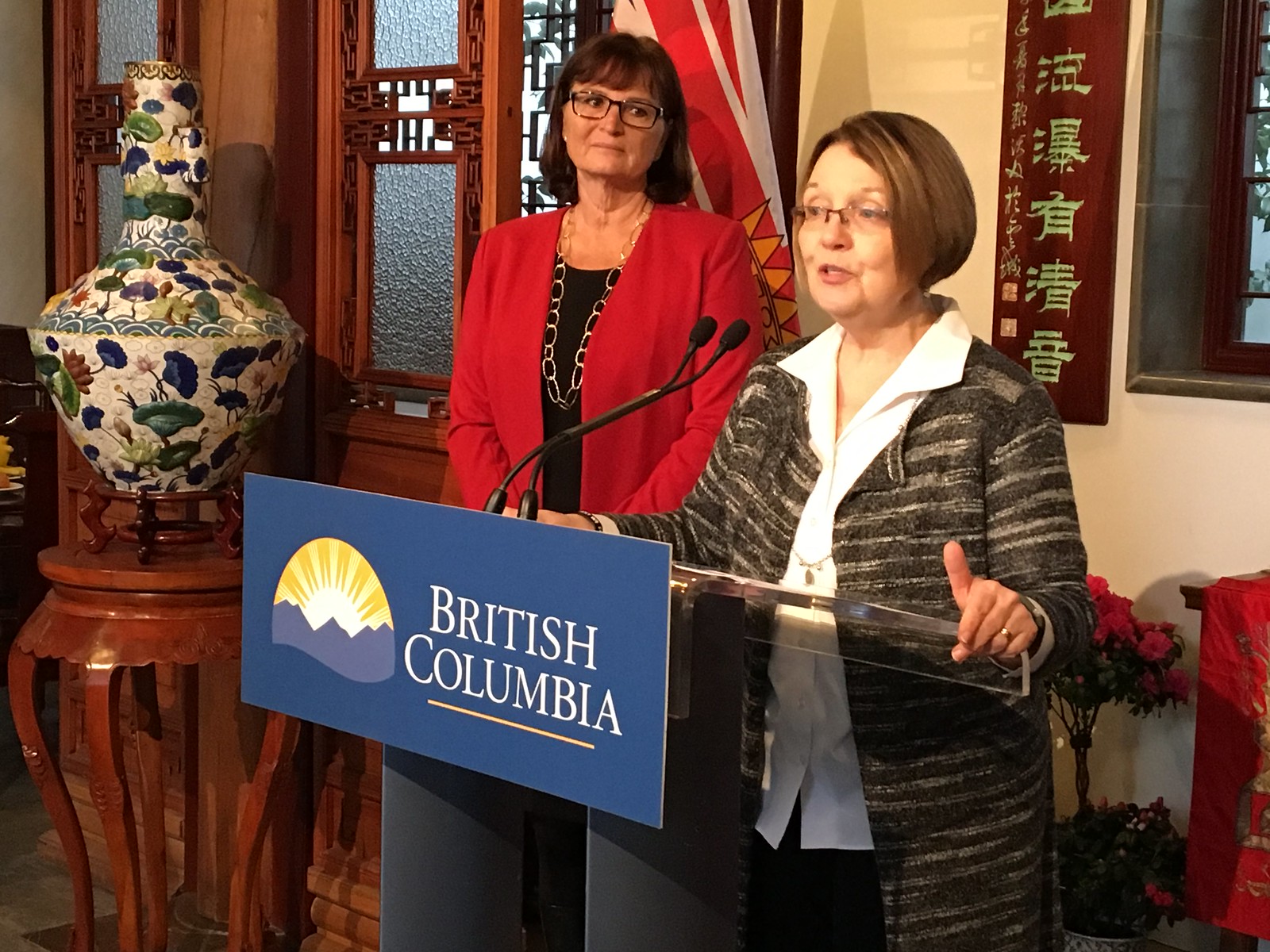The image depicts a press conference or event inside an old, ornate building. At the center is a clear plexiglass podium with two thin, navy beams and a blue sign that reads "British Columbia" in white letters, accompanied by an illustrated logo of mountains with a sunrise. A woman is standing behind the podium, speaking into a microphone. She is wearing a gray and beige striped sweater over a white collared shirt, has short hair, glasses, and her hands are resting on either side of the podium. To her left stands another woman, seen from the waist up, wearing a red blazer over a black shirt with a long silver chain necklace. She has dark shoulder-length hair and glasses, and is gazing at the speaker. The room features distinctive elements including a large, ornate vase with green, blue, and brown floral designs on an elegant wooden side table, a vertical sign with Asian lettering in green, and a partially visible BC flag adorned with red, white, and yellow patterns.